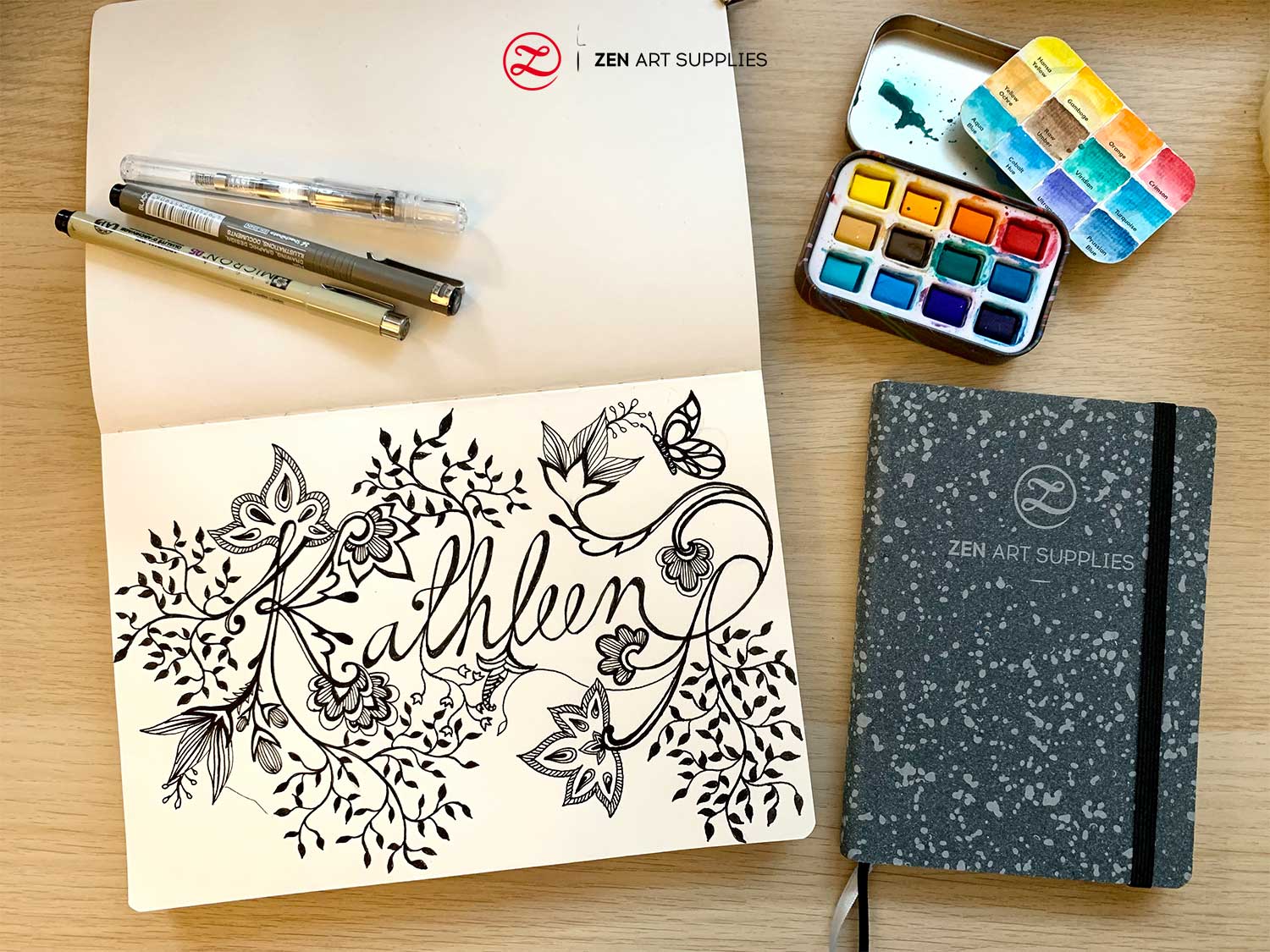This color photograph, taken from directly above in landscape orientation, captures an array of art supplies meticulously arranged on a light beige, blonde wood desk. Dominating the left side of the image is an open sketchbook, its blank white pages inviting creative exploration. The bottom half of the open pages features the name "Kathleen" elegantly written in black cursive, with the flourishes of the letters extending into intricate plant motifs, including flowers and ferns. Resting at an angle on the upper portion of the sketchbook are three closed black fine-tip pens.

To the right of the sketchbook lies an open watercolor tin, comprising twelve vividly colored paint pads arranged in three rows of four. The tin's lid serves as a makeshift palette, showing a mixture of blue paint, while a color swatch card, indicating various hues like yellow, orange, and blue, lies at an angle atop the tin. Below this, a closed gray notebook with speckled light gray accents is prominently displayed. The notebook's cover features a distinctive white "Z" encircled, with "Zen Art Supplies" inscribed in block lettering beneath it. A vertical black page holder secures the notebook, and a couple of ribbon markers peek out from its bottom left side.

Overall, the photograph embodies a serene and organized artistic workspace, perfectly capturing the essence of Photographic Representationalism, Realism, and Product Photography.